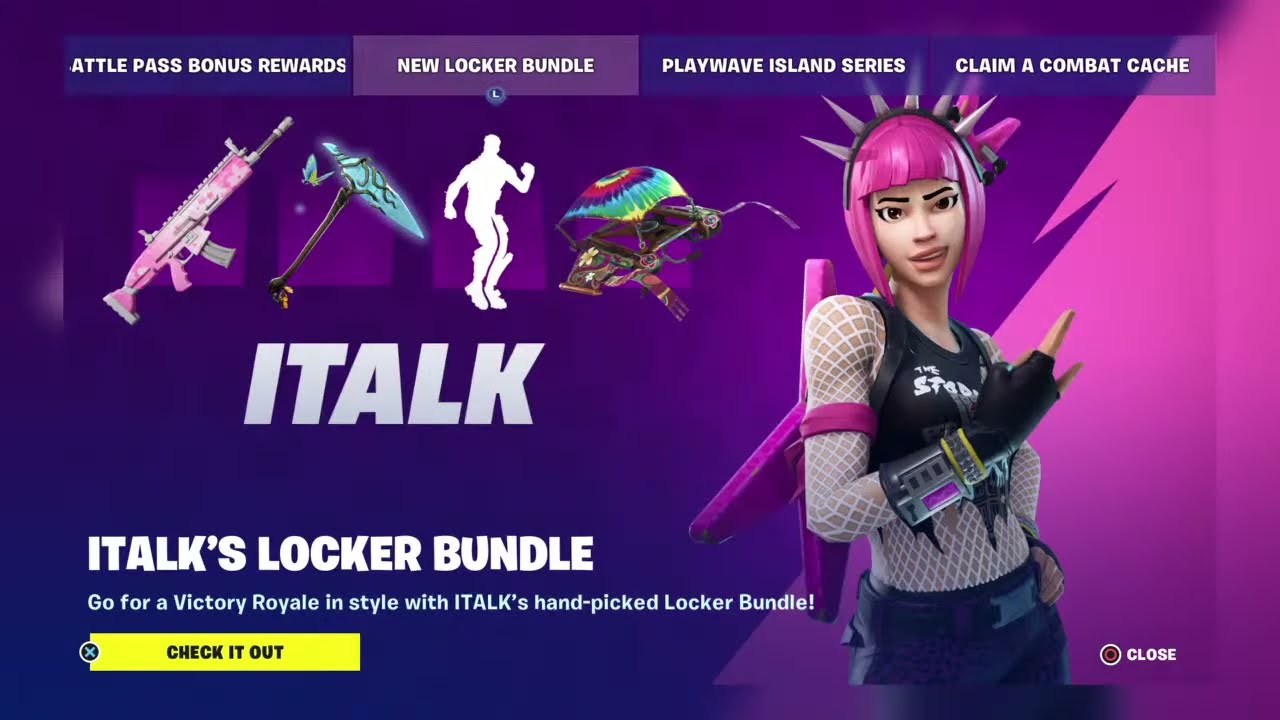The image is a screenshot of a video game promotion featuring a "Locker Bundle" with a vibrant purple background and a jagged dark pink protrusion resembling a half-silhouette of a pink Christmas tree in the right-hand corner. At the top, a banner displays four clickable options: "Battle Pass Bonus Rewards," "New Locker Bundle" (highlighted), "Play Wave Island Series," and "Claim a Combat Cache." Below these options are four icons: a pink and white cartoonish assault rifle, an axe with a shiny blue tip, a white silhouette of a man in a suit, and a hang glider with a tie-dye design. The text below reads "Italk" and "Italk's Locker Bundle. Go for a Victory Royale in style with Italk's Handpicked Locker Bundle." On the right side of the image is a digital character of a woman with pink hair and a headband with metal spikes. She is wearing a white fishnet shirt over a black crop top, complemented by black leather gloves and metal wristbands.